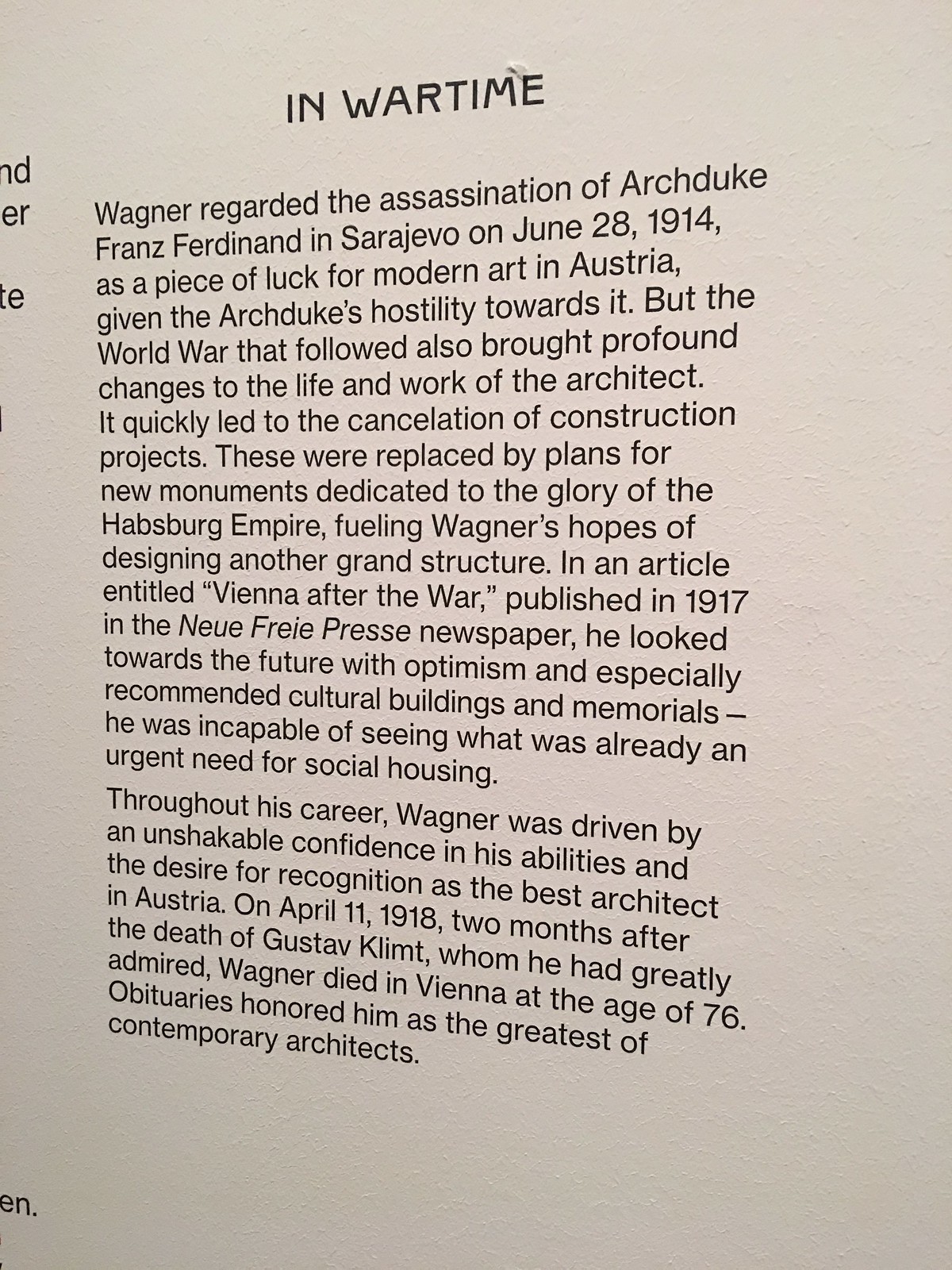The image depicts a museum sign on what appears to be cardboard, with a white-painted background and black text. The sign provides detailed historical information, stating that in wartime, architect Otto Wagner regarded the assassination of Archduke Franz Ferdinand in Sarajevo on June 28, 1914, as a piece of luck for modern art in Austria due to the Archduke's hostility towards it. However, the subsequent World War brought significant changes to Wagner's life and work, leading to the cancellation of construction projects and the shift towards designing new monuments dedicated to the glory of the Habsburg Empire. This change fueled Wagner's hopes of creating another grand structure. 

In a 1917 article titled "Vienna After the War," published in the New Free Press newspaper, Wagner optimistically advocated for cultural buildings and memorials, albeit neglecting the urgent need for social housing. Driven by a profound confidence in his abilities and a desire for recognition as Austria's foremost architect, Wagner continued his work until his death on April 11, 1918, two months after the passing of his admired contemporary, Gustav Klimt. Obituaries of the time honored him as the greatest contemporary architect.